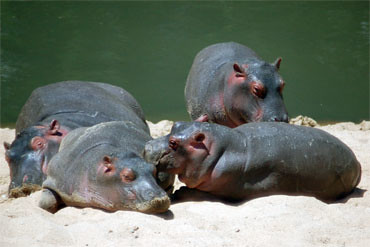This medium-sized, horizontally rectangular photograph features a charming scene of four juvenile hippos, predominantly gray with pinkish highlights around their eyes, ears, and shoulders. Three of these adorable hippos are lying down on a light sandy area in the foreground, with two appearing smaller and perhaps younger than the other two. Among these three, one is seen leaning its head on another who looks almost asleep. The fourth hippo, slightly larger, stands in the background. The upper half of the image reveals a body of dark green water, possibly indicating a river or similar habitat, contrasting with the sandy shore and suggesting a natural exhibit or safari environment. The general appearance of the hippos and their relaxed postures convey a serene and endearing atmosphere.